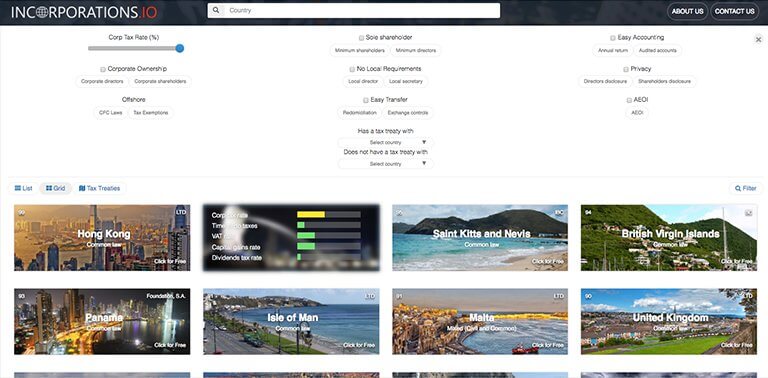The image features a webpage from the website "incorporations.io." At the top left corner, the website's name is prominently displayed. To the right of the logo, there is a search bar for user convenience. The main navigation menu includes options such as "Country," "About Us," "Contact Us," "Easy Accounting," "Minimum Shareholders," "Minimum Directors," "No Local Requirements," "Local Director," and "Local Secretary."

The webpage content includes references to different jurisdictions such as St. Kitts and Nevis, Malta, Isle of Man, Hong Kong, Panama, British Virgin Islands, and the United Kingdom, all of which are associated with common law. The visual design of the page incorporates a color scheme featuring shades of white, green, yellow, red, and brown, providing a vibrant yet professional appearance.